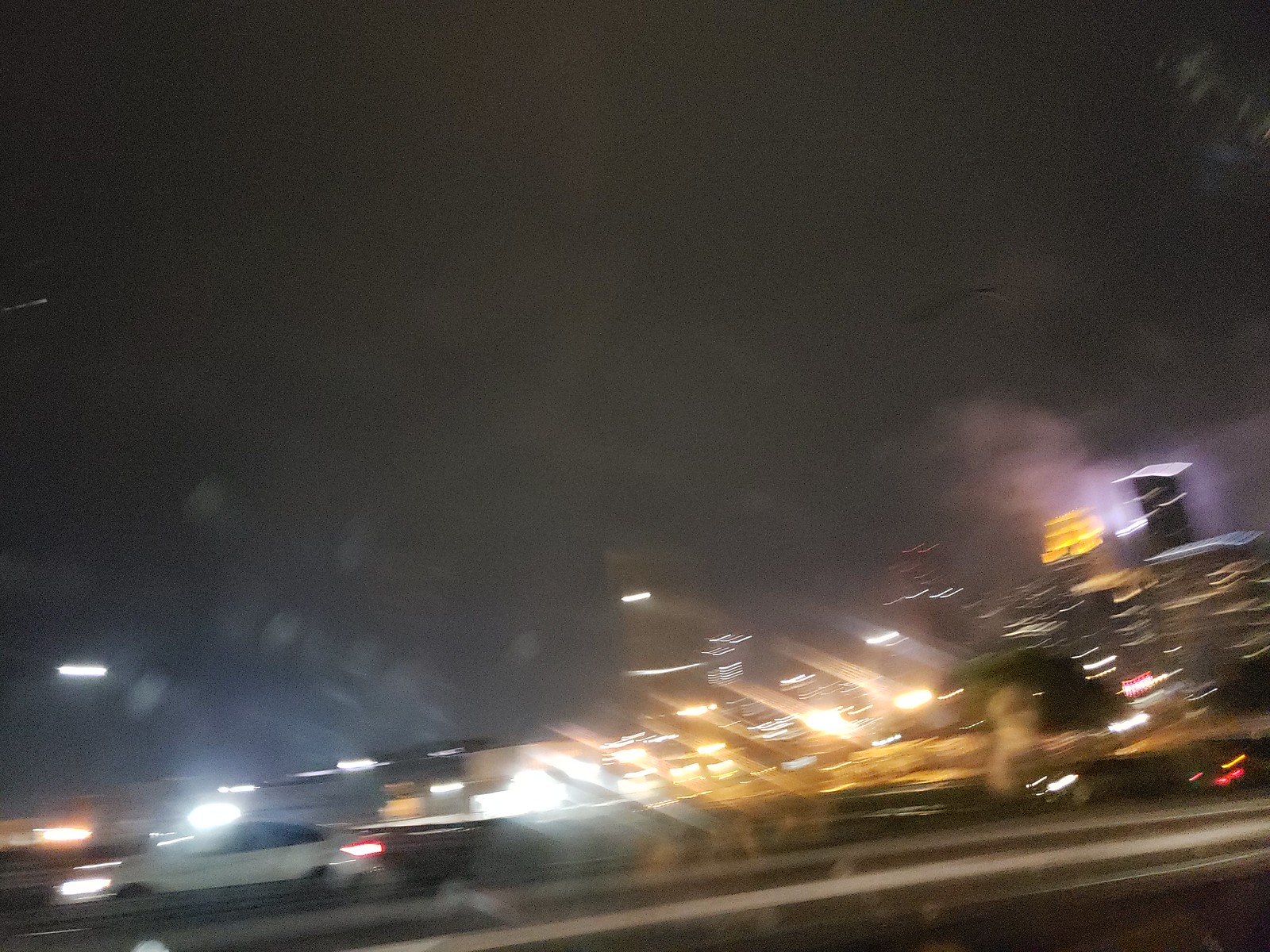This nighttime photograph appears to have been taken from inside a moving car on a freeway, with details made blurry due to motion. The image features a city skyline in the background, with numerous lit-up skyscrapers which create a sea of twinkling lights, further intensified by the reflections in the car's window. The sky is fully dark, indicating it is night. The city lights appear yellow in the windows, casting diffused reflections in various directions. In the foreground, there is an interstate highway. A white car with bright white headlights is visible in the lower left corner, accompanied by the red glow of its brake lights. Another, darker-colored car is visible farther back on the interstate, also with its headlights on. On the right side, behind the buildings, there is a prominent yellow illuminated area about an inch and a half high. The image quality is further compromised by fingerprints or possibly raindrops on the car window, adding to the overall blurriness and creating additional light distortions.